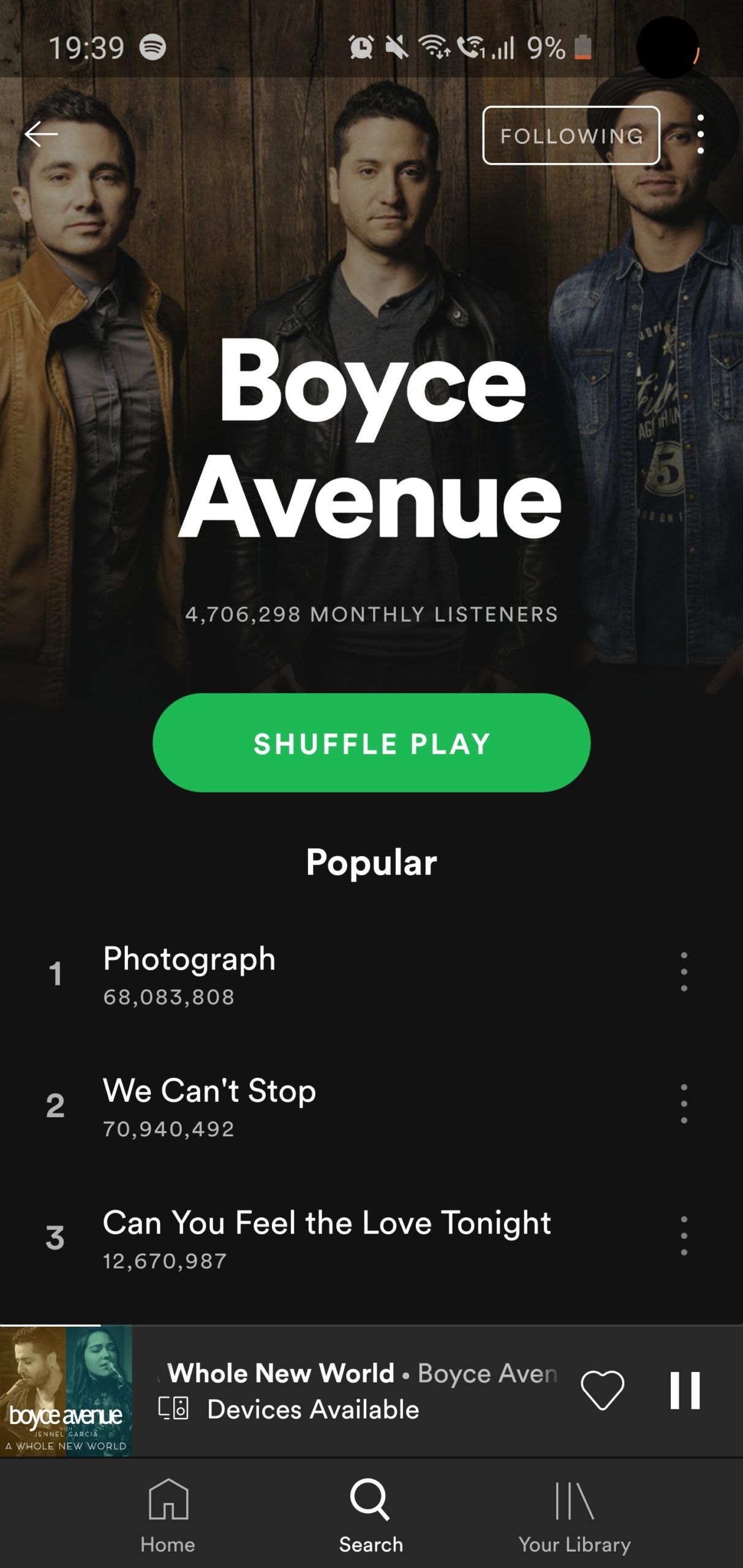**Detailed Caption:**
In this image, we see a smartphone screen displaying a music streaming app, which could be Spotify, Amazon Music, or Apple Music. The screen's time is set to a 24-hour format, showing 19:39 (7:39 PM). The phone's volume is muted, but its Wi-Fi connection is strong, and a call is in progress. The battery, however, is critically low at just 9%.

A popular band, Boyce Avenue, is prominently featured. Their profile image, showing three men, appears behind the band's name. Boyce Avenue boasts an impressive 4,706,298 monthly listeners, and the user is following them. The app interface suggests the option to shuffle play, although this button hasn't been pressed yet.

The band's top songs listed include "Photograph" as their number one hit, followed by "We Can't Stop" and "Can You Feel the Love Tonight." The currently playing song is "A Whole New World" by Boyce Avenue. An album icon is shown, but the heart icon to favorite the song has not been selected yet. The pause button indicates the song is playing.

At the bottom of the screen, the typical navigation icons for Home, Search, and Your Library are visible, offering the user easy access to other areas of the app.